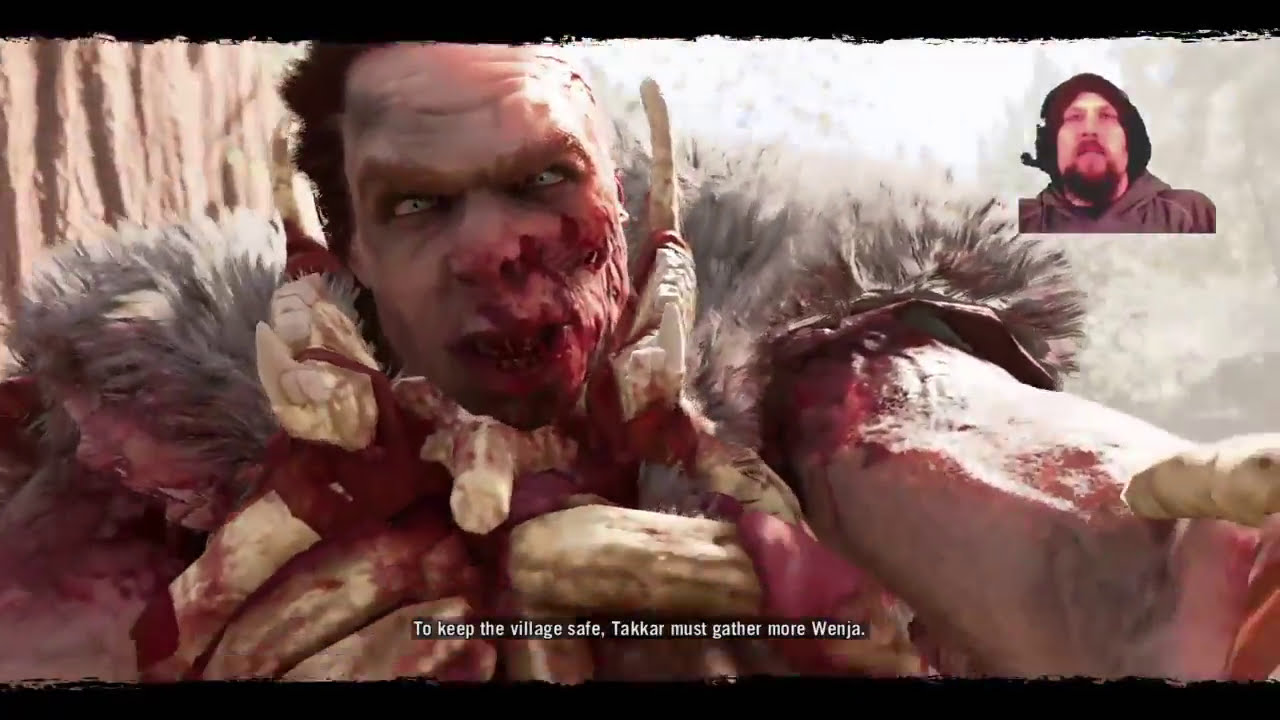This image captures a dramatic screenshot from a video game stream, highlighting a close-up of a Neanderthal-looking man who appears bloodied and intense. His wild, steel blue eyes stare straight into the camera, with blood smeared down the left side of his face and craggly teeth visible through his slightly open mouth. He wears a necklace of real bones and a fur collar, showcasing his muscled, bare arms in a chest-up view. His left arm extends outward, hinting at a "selfie" pose while his other hand is folded up in front of him. Text at the bottom of the screen reads, "To keep the village safe, Takkar must gather more Wenja." In the top right corner, the streamer is visible in a thumbnail; a middle-aged man with a thick goatee and mustache, donning a black Rastafarian hat and a brown hoodie, poised with a microphone setup. The scene immerses viewers in the raw intensity of the character and the gripping narrative of the game.